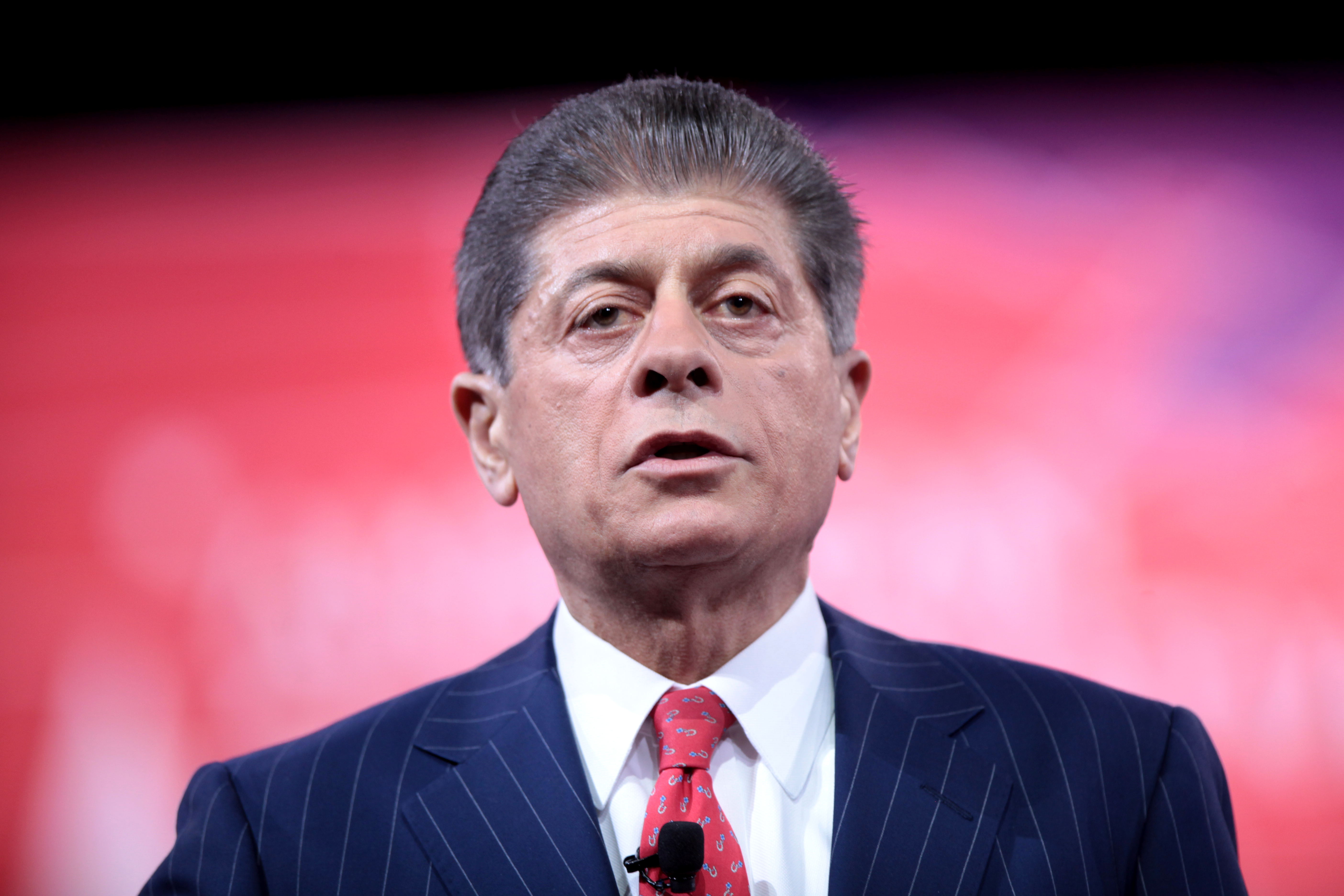This close-up photograph features a man centered in the image, looking directly forward. He has short, dark brown hair with touches of gray on the sides, neatly combed back. His head appears rounded on top. He is dressed in a dark blue suit jacket adorned with faint, possibly pinstripe patterns, though it's challenging to distinguish. Underneath, he wears a crisp white shirt paired with a pink tie that has some designs printed on it, to which a microphone is clipped. The photo is focused on him, while the background is beautifully out of focus, displaying a gradient of soft pink, white, and purplish hues, transitioning to black towards the top of the picture. The image is cropped at chest level, placing the man as the clear focal point against a subtle, muted backdrop.